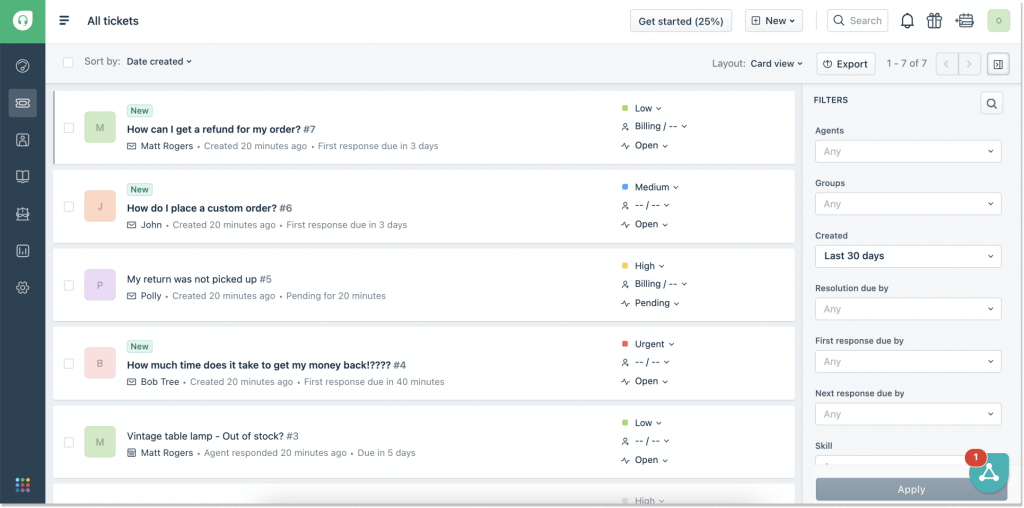This image is a detailed screenshot of a website dashboard laden with various elements and messages. 

On the left side, a dark blue vertical toolbar contains several icons, each representing different sections of the dashboard. From top to bottom, the icons include: a speedometer symbol, a ticket, a profile picture, a book, a character wearing glasses, a bar graph, and a cogwheel, which are all generic and indicative of typical dashboard functionalities.

The central portion of the screen displays a white header that reads "All Tickets," underneath which there are several interactive elements. Toward the top, there are statuses labeled "Get Started 25%" and "New." Adjacent to these are a search box, a bell icon (likely for notifications), a gift icon, and a calendar icon. Over on the far right of the screen, there's a mint green profile picture featuring the letter "O" in its center.

Directly below the "All Tickets" section lies a light gray header that includes options such as "Sort by," "Date Created," "Layout," and "Card View." Additionally, there's an "Export" button, and to its right, pagination indicators "1 to 7 of 7" alongside gray arrows pointing left and right for navigation.

Following this header, the main content section lists five distinct messages, each contained within a white box separated by gray dividers. The first message, labeled "New," reads: "How can I get a refund for my order, number seven." This ticket was created by Matt Rogers 20 minutes ago, with the first response due in three days. It is marked low priority, highlighted by a green box, and categorized under "Billing" with a person icon. The status is "Open," indicated by a chart icon.

The second message, also marked "New," queries: "How do I place a custom order, number six." Created by John 20 minutes ago, this ticket too has the first response due in three days. It holds a medium priority status, denoted by a blue box, and has a placeholder for specific categories (represented as "2 dashes / 2 dashes") alongside a person icon and a status of "Open" with a chart icon.

Similar formatting and details apply to the three additional messages listed beneath these, each encapsulated within their own white boxes and reflecting the workflow of the support or ticketing system the dashboard is managing.